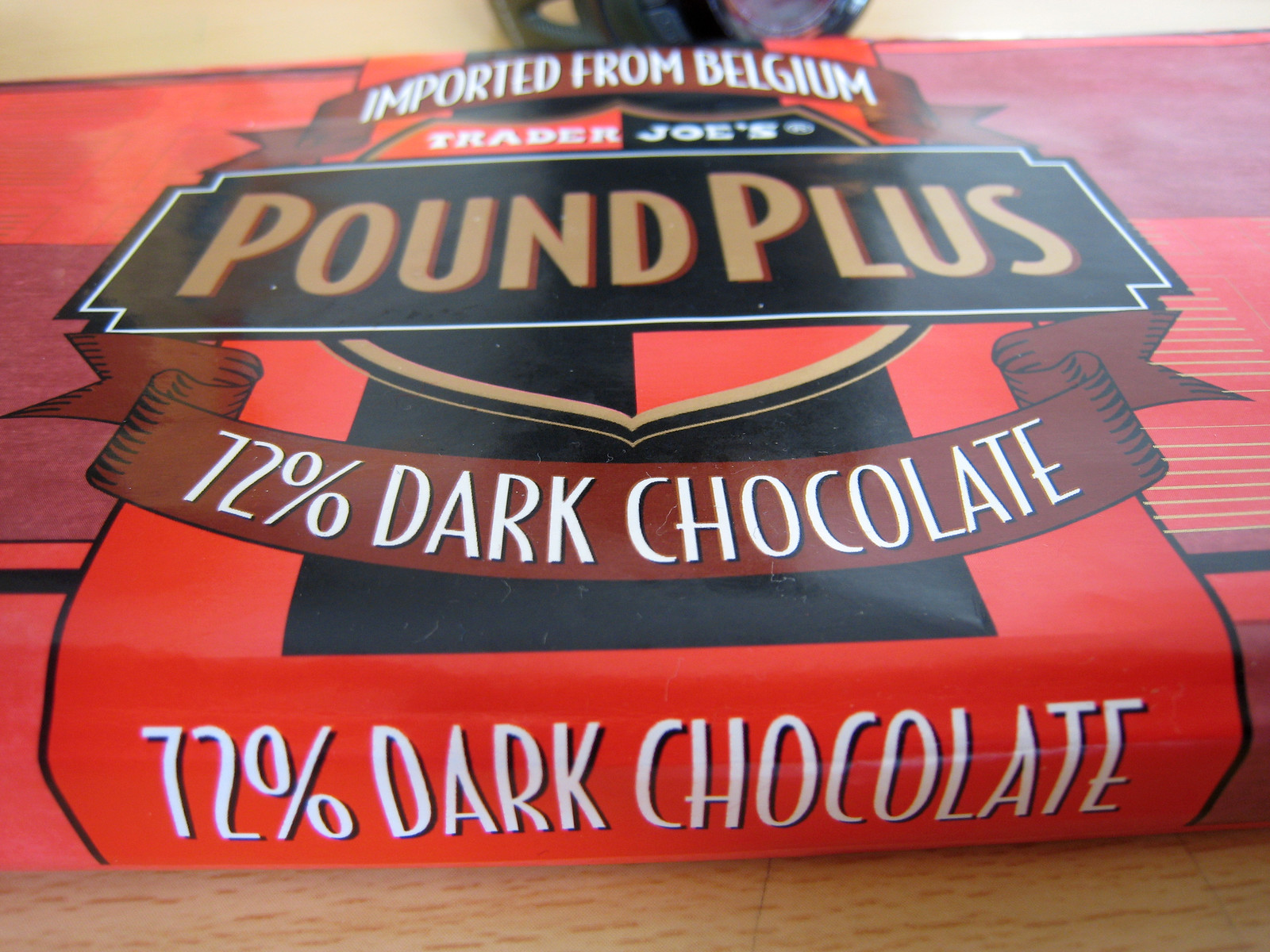The image depicts a close-up of a chocolate bar package, prominently featuring shades of red and brown, photographed on a wooden surface. The package's design is intricate, with several noteworthy elements. At the top of the red package, against a blue banner, the text "Imported from Belgium" is written in white. Below this, a coat of arms design is central, with "Trader" inscribed in white on the red portion and "Joe's" in white on the black portion of the shield. Beneath this shield, a black, rectangular label contains the words "Pound Plus" in bold brown lettering. Another feature of the package is a brown banner that declares "72% Dark Chocolate" in white, which also appears along the bottom edge of the package. The borders of the package reiterate "72% Dark Chocolate" in white against a red background. This detailed packaging design marks it clearly as a Trader Joe’s product, specifically highlighting its Belgian origins and high cocoa content.